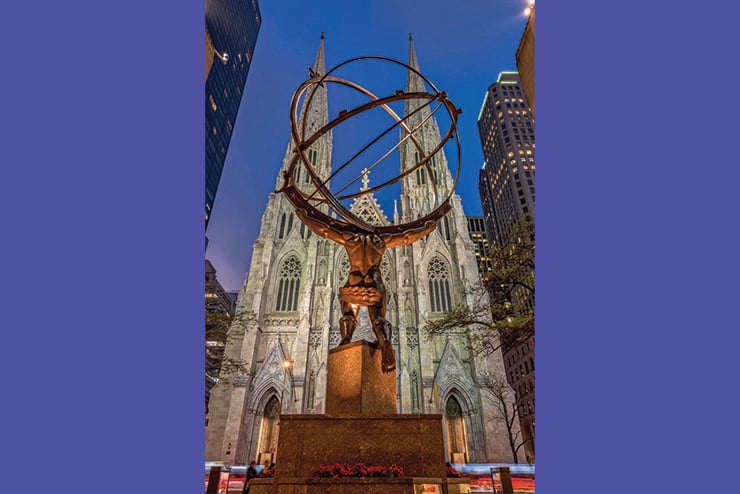The image depicts a detailed color photograph with large blue borders on the left and right, focusing on a bronze statue of a man resembling Atlas. The statue is situated on a well-defined base comprising a brown pedestal and a smaller rectangular platform. The statue, viewed from behind, shows Atlas with outstretched arms holding a large gyroscope-like circular metal structure on his back, with his left foot positioned firmly on the base and his right leg hanging down.

In the background, prominently featuring a magnificent white stone cathedral, the scene is framed by city skyscrapers extending off the image's edges. The cathedral, embodying European church architecture, boasts two high steeples on either side and a smaller central steeple topped with a cross. The structure is adorned with two entrances and intricate secret window designs, with noticeable cross motifs. Surrounding the base of the statue are vibrant flowers, adding color to the setting. The scene is captured under a deep blue evening sky, with lights illuminating the top right of the buildings, enhancing the overall ambiance of the photograph.